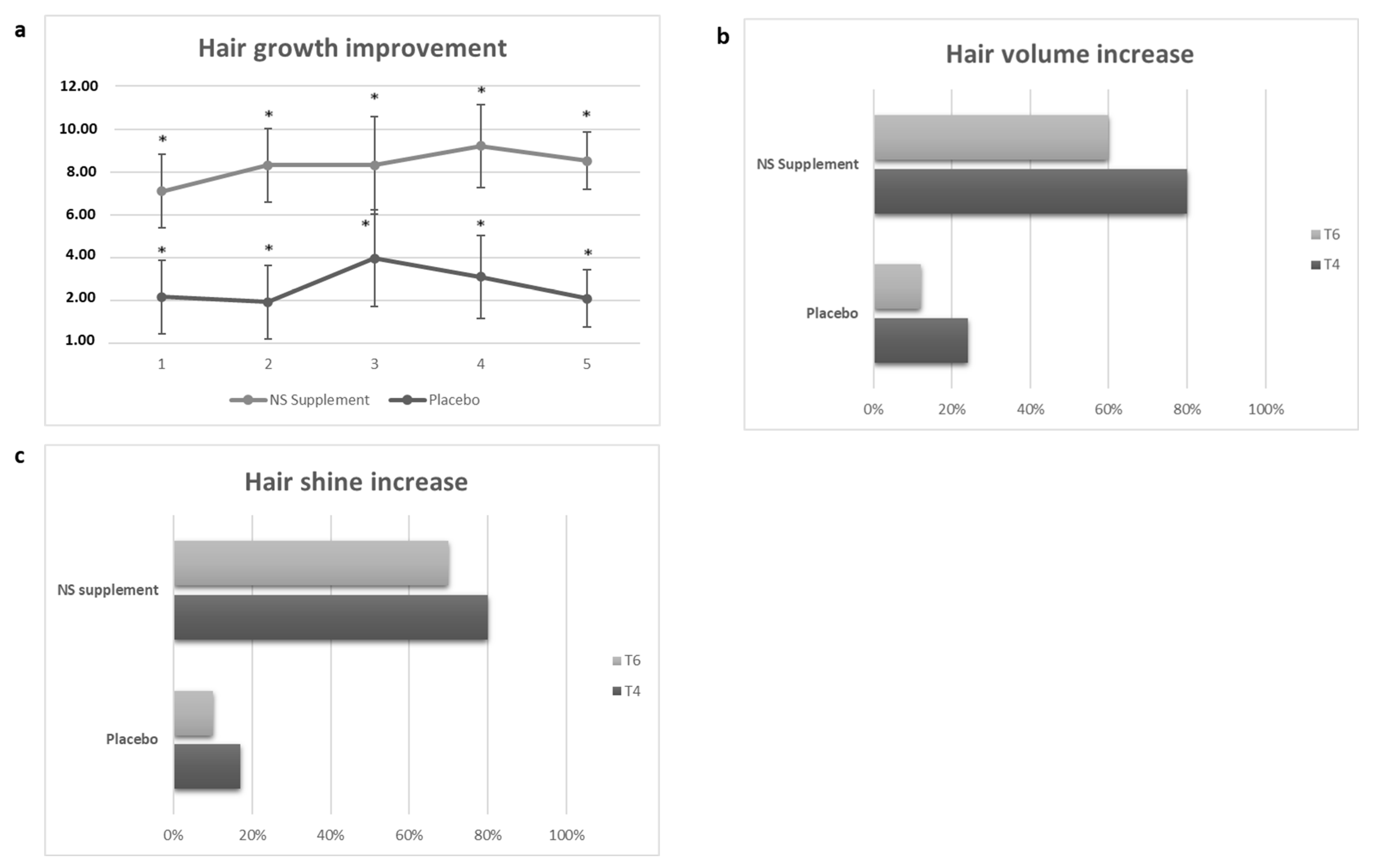This black and white image presents three distinct graphs, each enclosed in a light gray border and identified by labels A, B, and C in the top left corner of each section. The lower right quadrant of the image is intentionally left empty. 

Graph A, situated in the upper left, is a line graph titled "Hair Growth Improvement." It features two lines—a light gray line representing the NS supplement and a dark gray line for the placebo. The y-axis is numbered from 1 to 12, and the x-axis from 1 to 5, depicting different time points. The data is complemented by a key beneath the graph.

In the upper right, Graph B is a bar graph titled "Hair Volume Increase." It showcases NS supplement and placebo treatments with light gray and dark gray bars, respectively. The x-axis marks percentage values from 0 to 100 in increments of 20. The light gray bars (T6) and dark gray bars (T4) indicate specific time intervals, showing NS supplement percentages at approximately 60% and 80%, and placebo values at roughly 15% and over 20%.

Graph C, in the lower left, is similarly a bar graph, labeled "Hair Shine Increase." This graph also distinguishes between NS supplement and placebo using light gray (T6) and dark gray (T4) bars. The percentages at T6 and T4 for NS supplement are 70% and 80%, respectively, while the placebo reaches 10% at T6 and 18% at T4.

Each graph effectively highlights the comparative performance of the NS supplement versus the placebo across different measures: hair growth, volume, and shine.